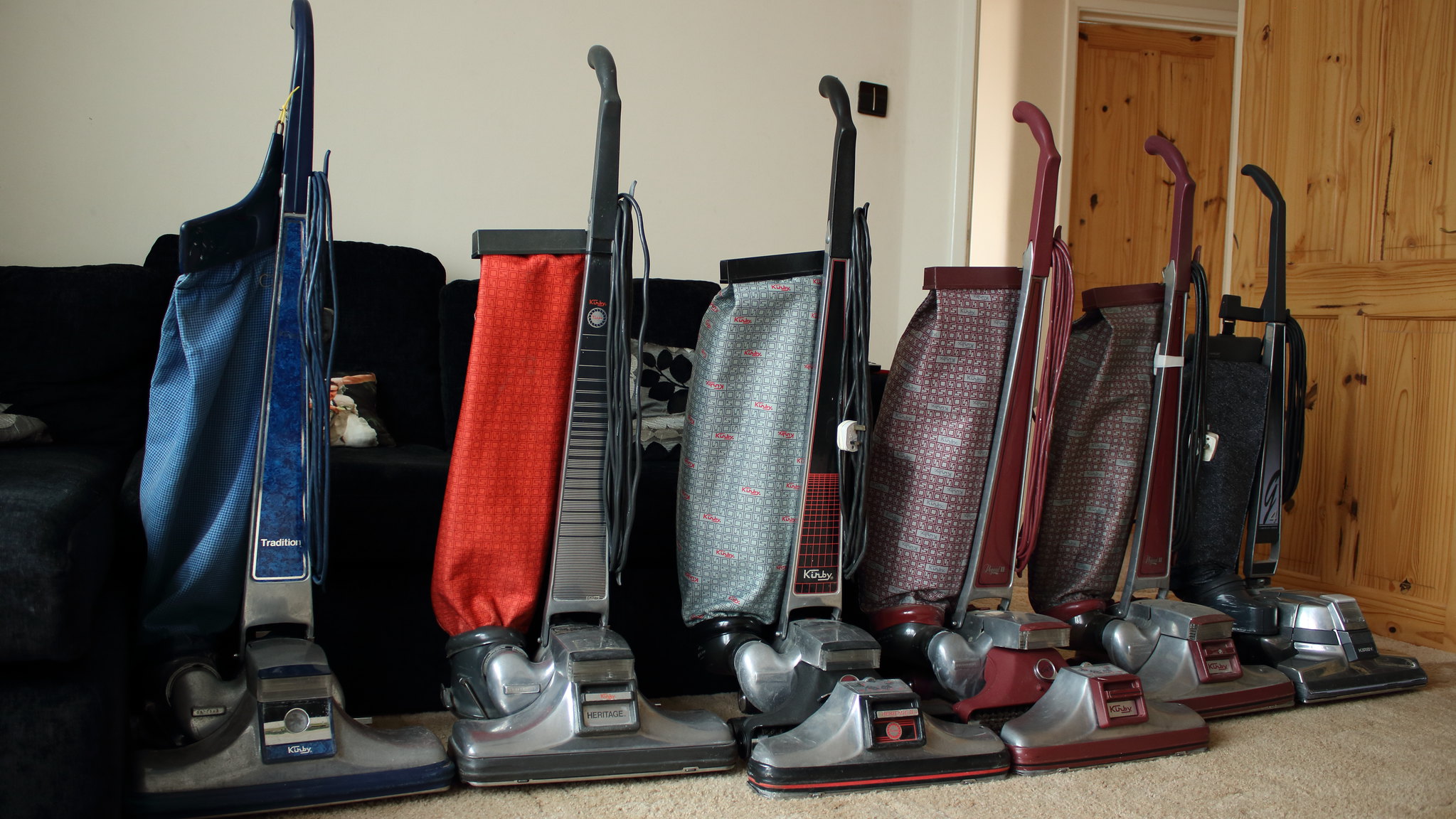The photograph captures a room filled with six vintage vacuum cleaners, each showcasing a distinct, old-fashioned design reminiscent of the 1950s or 60s. The vacuum cleaners are lined up against a backdrop of beige carpet and light blue walls with knotty pine shelves reaching from floor to ceiling. The first vacuum on the left features a navy blue bag and a black handle with a black base. Next to it is a vacuum with a black handle, a black bag adorned with white stripes, and a silver detail at the base of the bag. Following that, there's a vacuum with a black handle and a gray bag decorated with small red floral patterns, along with a primarily silver base accented with black and red. The subsequent two vacuums are practically identical, both sporting burgundy handles, bases, and caps, with a long, silver, and burgundy bag. The last vacuum on the right appears to have a black handle, a black bag, and a silver and black base, though it's partly obscured, making details hard to discern. The vacuums are meticulously arranged, possibly part of a collection or for sale, and to the far right of the image, a closet can be seen in the background. Additionally, a sofa with throw pillows is partially visible behind the vacuums, adding to the room's cozy atmosphere.